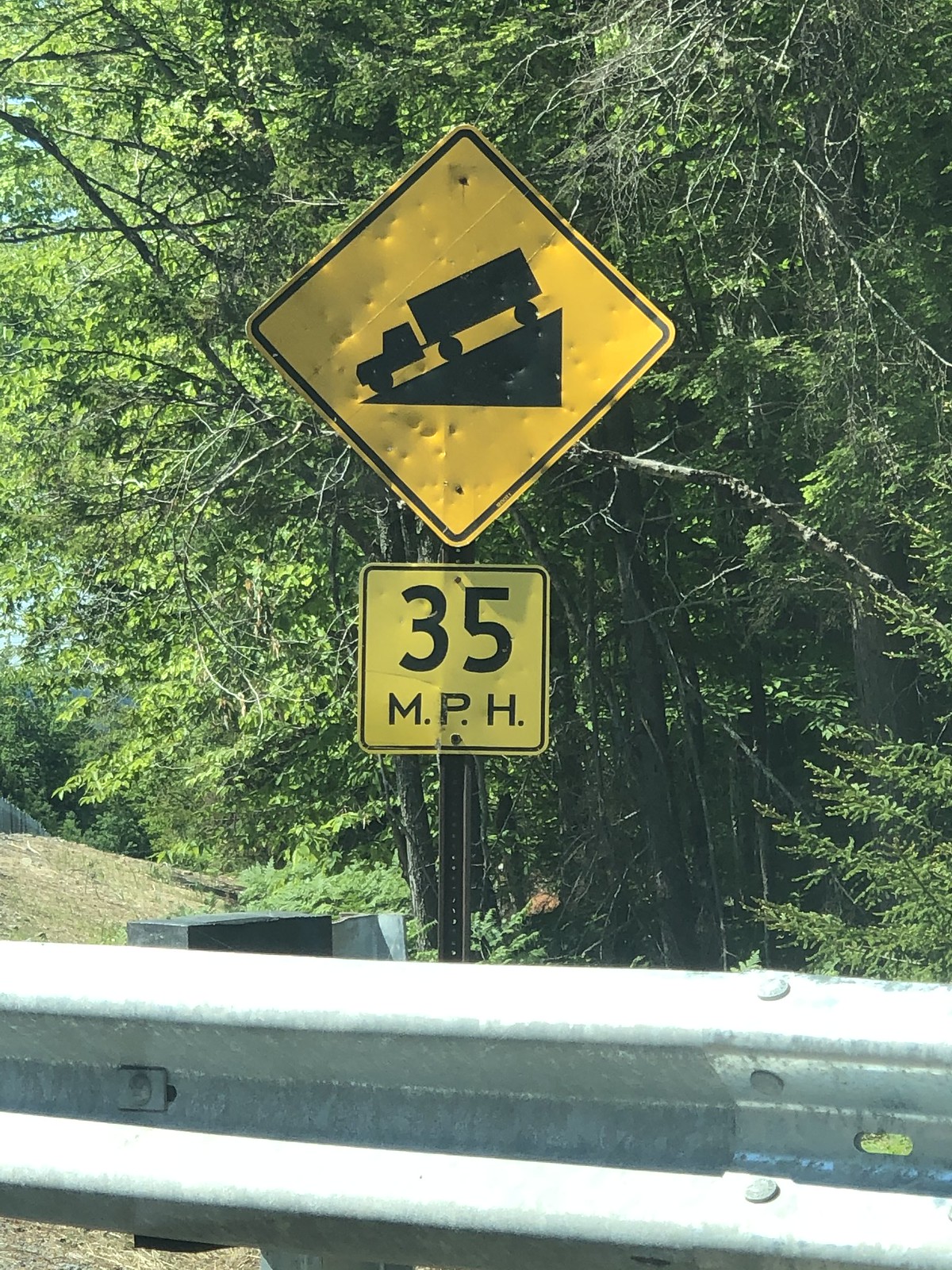A photograph captures a roadside scene on a sunny day. The clear blue sky peeks through a dense collection of trees, some of which exhibit bare branches while the majority are lush with green leaves. In the foreground, a gray metal guardrail lines the road, providing safety for vehicles. The focal point of the image is a distinct road sign. The sign is square-shaped but oriented in a diamond position, with points at the top and bottom. The sign features a black triangle with a truck descending a slope, symbolizing a steep grade. Below the triangle, the text "35 M.P.H." is prominently displayed. The entire sign, including the cautionary symbols and text, is rendered in black on a bright yellow background.